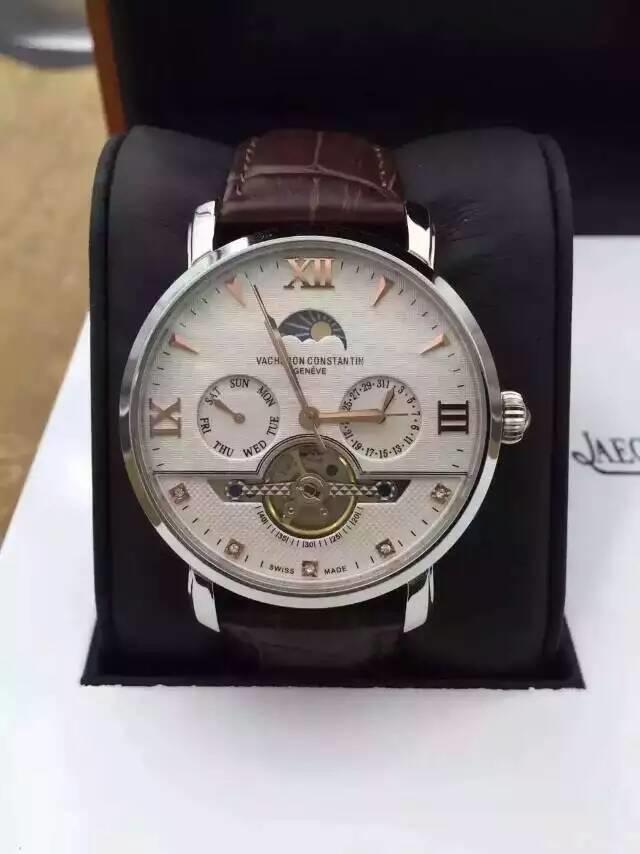The image shows a meticulously designed watch encased in its display box. The watch is set against a black stand, and the band is crafted from dark chocolate brown leather, exuding elegance. The outer border of the watch is silver, while the face is off-white. Notably, the Roman numerals marking the hours 12, 1, 2, 3, 9, 10, and 11 are rendered in a golden hue, with the remaining numerals indicated by what resembles tiny diamonds. The watch hands are also gold, enhancing the luxury aesthetic. Within the dial, the brand name can be faintly discerned as "BACH Constantin," with "Geneva" inscribed beneath it. Additionally, the watch features a visible gear mechanism and two smaller dials; one on the left shows the days of the week, currently pointing to Saturday, and another on the right likely indicates the date. The background reveals a brownish, possibly wooden floor, and a chair with a black seat and dark brown border, which frames the luxurious timepiece in a sophisticated indoor setting.